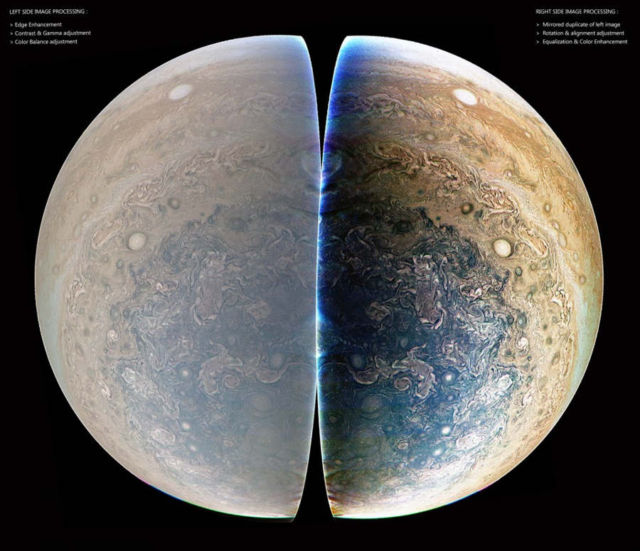This image features a highly magnified, cross-sectional view of a spherical object, divided into two symmetrical halves against an entirely black background. Each half displays distinct, intricate patterns suggestive of geological textures. Starting from the outermost areas, there's an off-white layer gradually transitioning into lighter and then darker brown stripes, reminiscent of rocky surfaces. Moving inward, the core features vibrant hues of aqua and dark green, possibly indicating water or mineral deposits. 

The halves appear slightly misaligned, implying the object was bisected and then rejoined imperfectly. This composition could result from comparing different imaging techniques or lenses, as suggested by the subtle differences in pattern clarity and color saturation. Indeed, there are small, barely legible annotations in the upper left and right corners of the image that read "left view image processing" and "right view image processing," which potentially provide clues to the visual discrepancies. The image evokes a planetary cross-section, though it distinctly lacks the familiar features of Earth's moon, hinting at a more exotic celestial body.